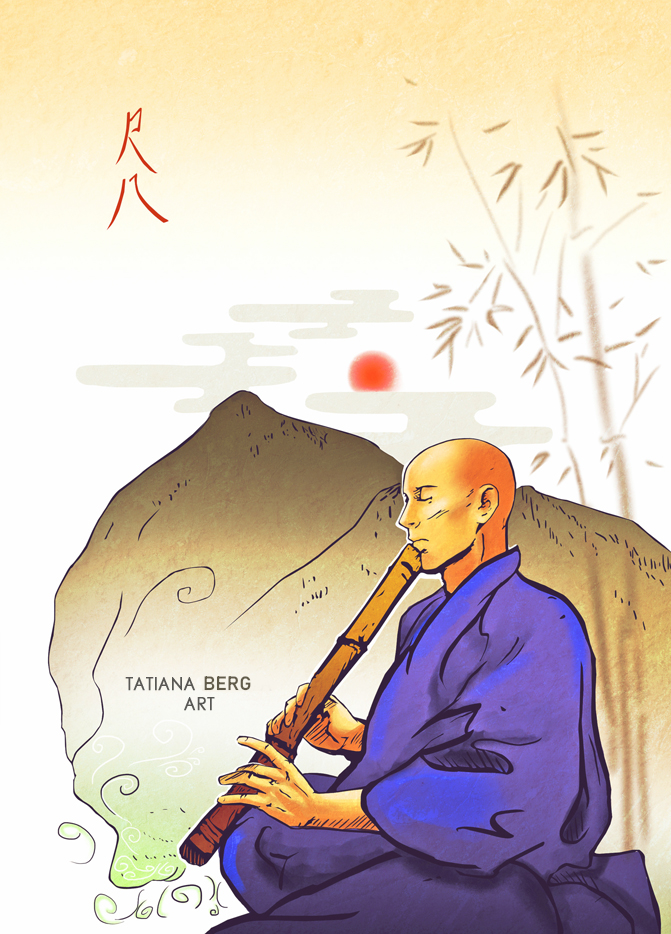In this evocative painting, a man, possibly a monk, is depicted seated on the ground next to a large rock outcrop. He holds a unique woodwind instrument to his mouth, with both hands perfectly positioned for playing. The man is clad in a flowing robe that shades from blue to bluish-purple, and he is bald, emphasizing his serene, contemplative demeanor. The background features delicate, faint imagery of trees or bamboo, creating a tranquil, natural setting. Intriguingly, the top left corner of the painting includes script, likely in Mandarin, although its meaning remains unknown. The artist's signature, "Tatiana Berg," is inscribed on the rock beside the man, followed by the word "Art." This detailed and intricate portrayal offers a glimpse into a peaceful moment of musical meditation.